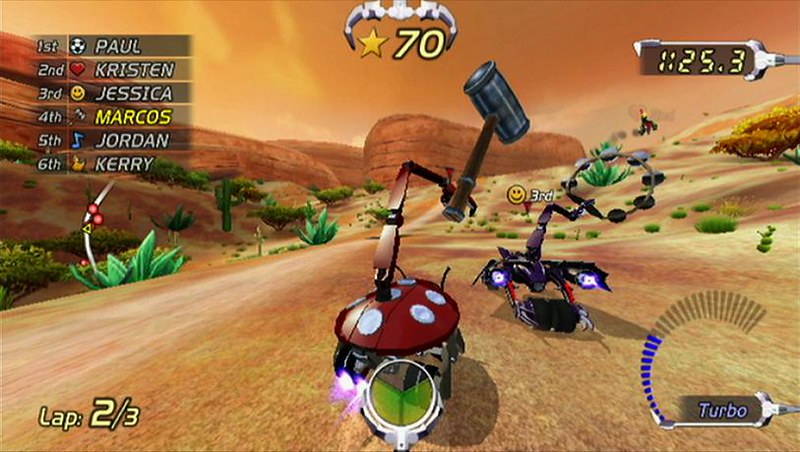This screenshot captures an intense moment of gameplay in a desert-themed racing game featuring robots. The vibrant desert setting is enriched with terracotta-colored canyons and scattered green cacti. On the left side of the screen, player names and their corresponding icons are listed alongside their positions: 

- Soccer ball, Paul (1st)
- Heart, Kristen (2nd)
- Smiley face, Jessica (3rd)
- Gavel, Marcos (4th)
- Music note, Jordan (5th)
- Duck, Carrie (6th)

At the top center, a gold star icon with the number 70 is prominently displayed. To the right, yellow numbers reading "1.25.3" are shown. In the race, one robot stands out with a bronzy arm resembling a hammer, a red ladybug-like shell adorned with white circles, gray wheels, and green accents at the back. Another robot, with sleek black, blue, and red coloring, features a circular attachment. Lower down the screen, 'Turbo' is written in blue alongside an arched blue line, while "Lap 2 of 3" is indicated on the opposite side.